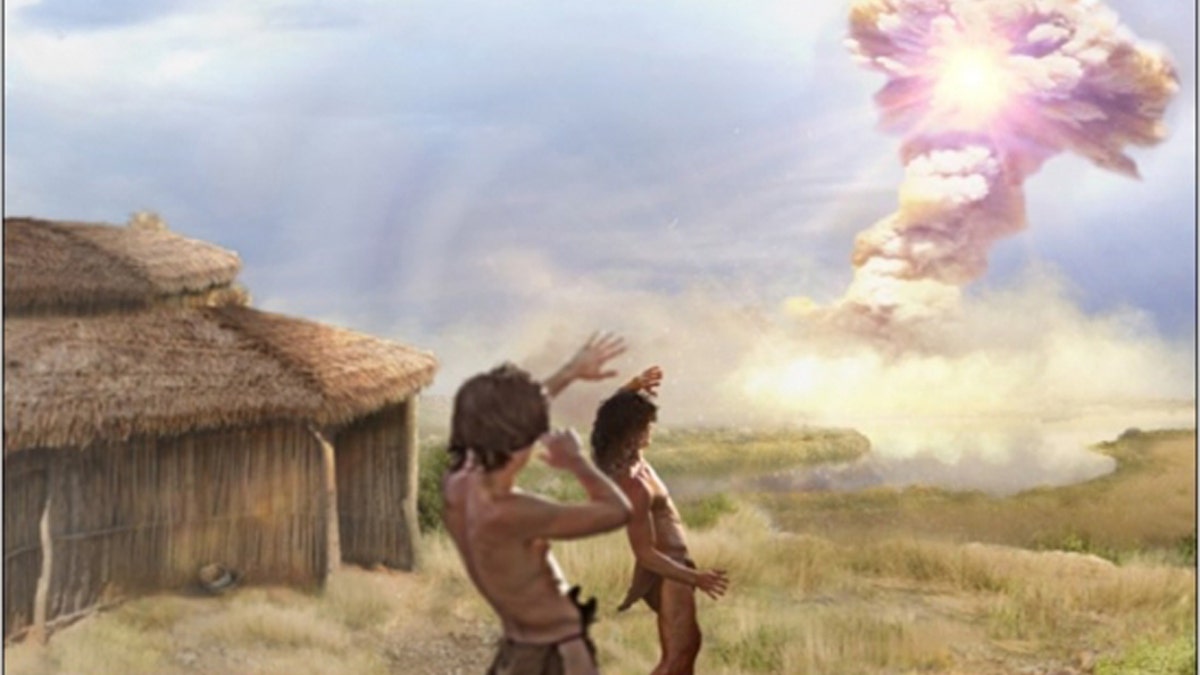The image depicts a painting, possibly AI-generated, of a nuclear explosion occurring in the distance under a blue sky with scattered clouds. Two young, ancient-looking boys, resembling cavemen, stand in a vast expanse of light grassy fields, both shielding their eyes from the glaring light of the explosion with their left hands. One boy, with shorter, shaky brown hair, also raises his right hand to his face, while the other boy, with longer, curlier hair, lets his right hand rest at his side. They are both shirtless, wearing only loincloths. Nearby, on the left, stands a hexagonal hut made of straw and grass, with a bull resting against its wall. The explosion's dramatic display features a white cloud of smoke rolling upwards, transitioning through shades of purple and gold, culminating in a brilliant, bright core. The powerful blast sends debris and smoke rolling toward the boys, illustrating a stark and surreal contrast between primitive life and catastrophic destruction unfolding before them.